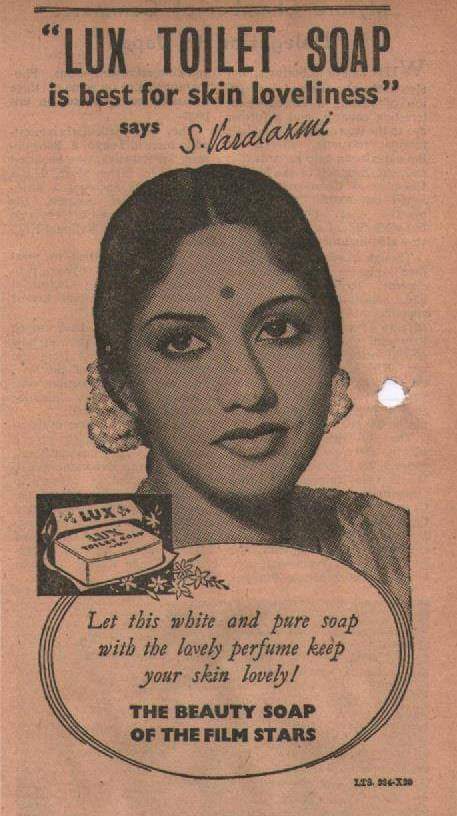This is a vintage advertisement for Lux Toilet Soap featuring a grayscale image of an Indian woman at the center. She has a red dot (bindi) on her forehead and exudes a serious expression, looking straight at the camera. She has dark hair that appears pulled back, possibly held by a fancy headband, and wears makeup. The ad showcases a classic 1940s-1950s design style, reminiscent of old school newspaper artwork.

At the top of the ad, there is text in quotation marks reading, "Luxe Toilet Soap is best for skin loveliness," attributed to S. Farrah. The woman’s image has a notable hole to the right side of her face, adding to the vintage feel of the ad. Below her face is an illustration of a box of Lux Soap with the lid open. Surrounding the central image is promotional text in tan, black, and gray colors which says, "Let this white and pure soap with this lovely perfume keep your skin lovely, the beauty soap of the film stars," reinforcing the soap's status and elegance. The overall composition and color palette, including tan, black, and gray hues, emphasizes the ad's antique charm while the soap's placement in an open box at the bottom left adds a tactile element to the visual.